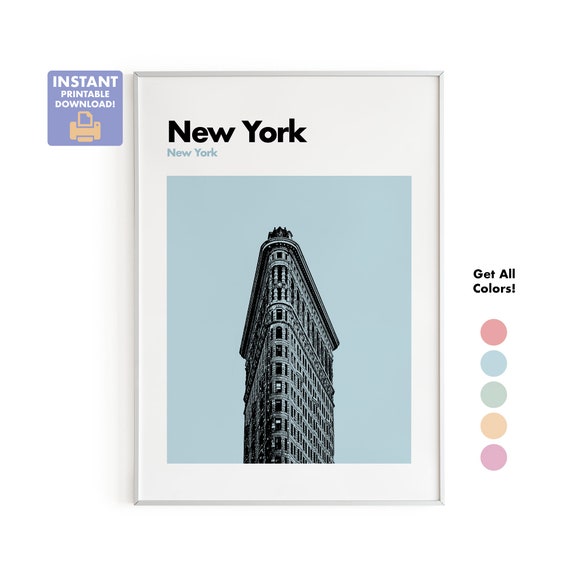This image is an advertisement for an instant printable download, featuring a framed poster with a white background for clean presentation. Within the white frame, at the top, the poster has the text "New York" in black, followed by "New York" in smaller, light blue text underneath. The centerpiece is an artistic rendition of the iconic Flatiron Building in New York, depicted in a light blue hue. The simplistic artwork adds an elegant touch without cluttering the background, which remains a generic, light blue sky. 

In the top left corner outside the frame, there is a rectangular logo with a light blue interior that reads "Instant Printable Download" in white text above a small printer icon. The bottom right corner of the image highlights the availability of multiple color options for the poster, listing them in black text as "Get All Colors." Displayed below are five pastel color samples: light red, light blue, light green, light orange, and a light pinkish color. The overall aesthetic of the advertisement emphasizes a minimalistic and versatile design suitable for various color preferences.